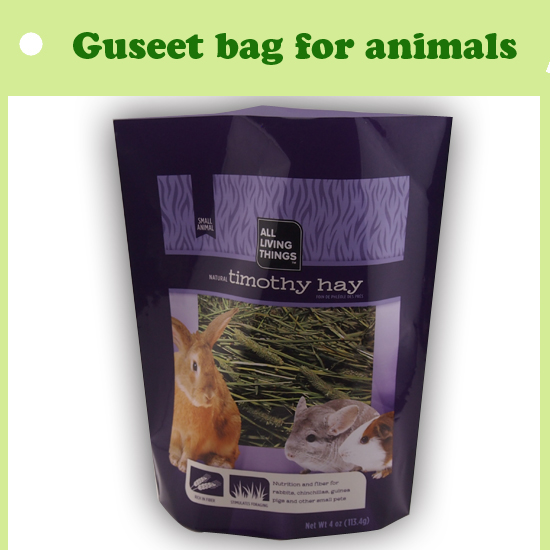The image depicts part of an advertisement featuring a purple bag of Natural Timothy Hay, designed for small animals, from the brand All Living Things. The bag is set against a white background with a prominent lime green border that thickens at the top, where in darker green text it reads "Guseet Bag for Animals" (G-U-S-E-E-T). The bag itself is slightly open at the top, displaying a product tag labeled "Small Animal." The main section of the bag showcases a photograph of Timothy Hay, accompanied by images of a brown rabbit on the left, a gray chinchilla in the center, and a white and tan guinea pig on the right. Additionally, there is a small, unreadable white banner at the bottom of the bag. The top left corner of the image includes a white hole punch. The overall presentation and photography suggest the image is intended for a website or catalog advertisement.